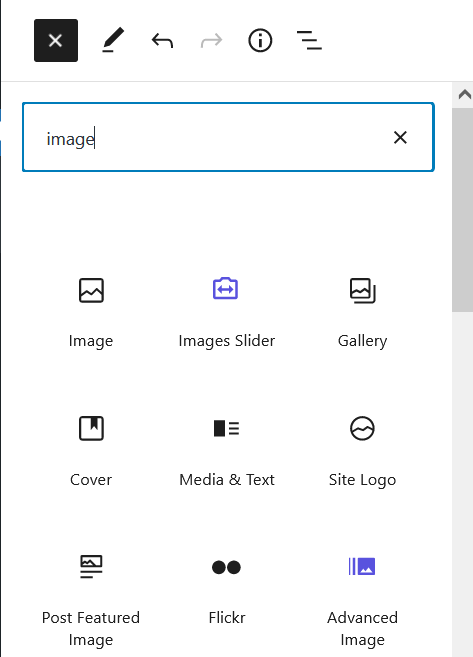This image appears to be a screenshot taken from a smartphone displaying a mobile app interface for searching and organizing media. The screen is divided into three rows, each containing three icons representing different media management functionalities. These icons are text-based with simplistic drawings.

At the top of the screen, there is a teal-outlined search box, with the word "image" typed into it. Situated above this search box are several icons: a white 'X', a black box, an edit icon, a back arrow, an inactive forward arrow, an information icon within a circled "i", and a three-line menu icon for additional options.

The three rows of app functionalities are organized as follows:

- **First Row:**
  - **Image**: Simple drawing and text.
  - **Image Slider**: Simple drawing and text.
  - **Gallery**: Simple drawing and text.
  
- **Second Row:**
  - **Cover**: Simple drawing and text.
  - **Media and Text**: Simple drawing and text.
  - **Site Logo**: Simple drawing and text.
  
- **Third Row:**
  - **Post Featured Image**: Simple drawing and text.
  - **Flicker**: Simple drawing and text.
  - **Advanced Image**: Simple drawing and text.

The layout and icons suggest an organized yet minimalist approach to navigating through various media and text functionalities available in the app. This intuitive design aims to streamline user interaction by providing clear and straightforward options.